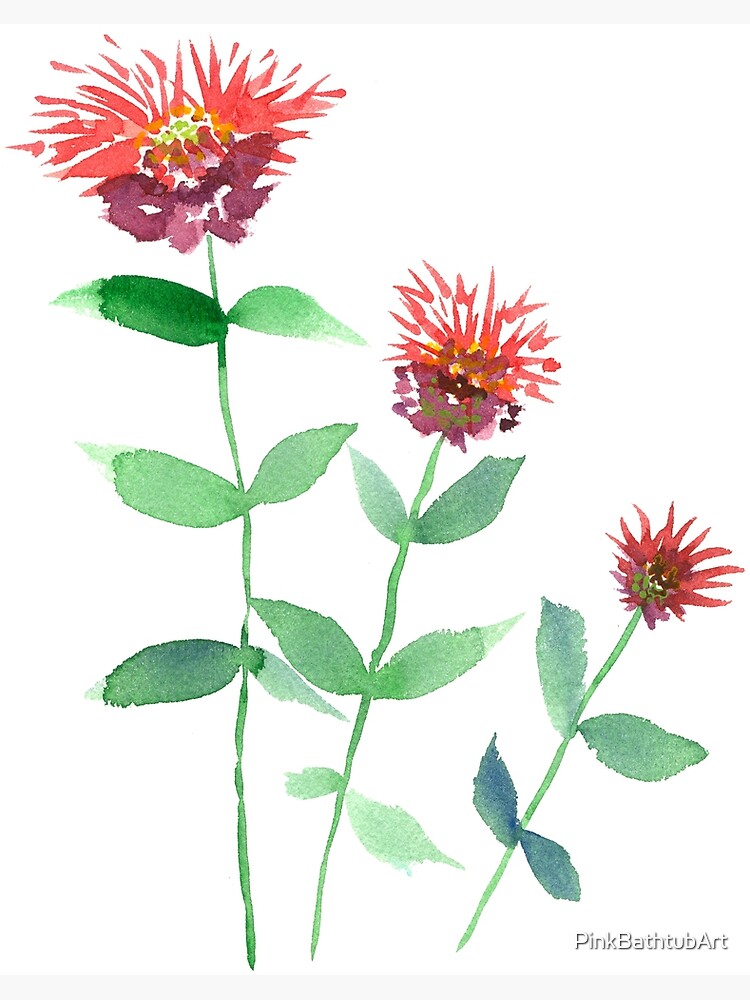This up-close scientific watercolor painting depicts three stages of a flower's growth from right to left, showcasing varying heights and detailed botanical features. Set against a white background, each flower has a green stem and a combination of blue and green leaves, with the tallest on the left having six leaves, the middle one also sporting six leaves, and the smallest on the right displaying four leaves. The flowers' petals are beautifully rendered with pink, red, and violet hues, starting from a dark reddish-burgundy at the tips to lighter shades towards the center. The yellowish pistils are accented with orange and yellow dots. The artwork, descriptively labeled "Pink Bathtub Art" in the bottom right-hand corner, suggests it could be ideal for bathroom decor. The flowers visually narrate a progression: the smallest flower on the right appears partially blooming, the medium one in the middle shows further blossoming, and the tallest on the left is in full bloom.